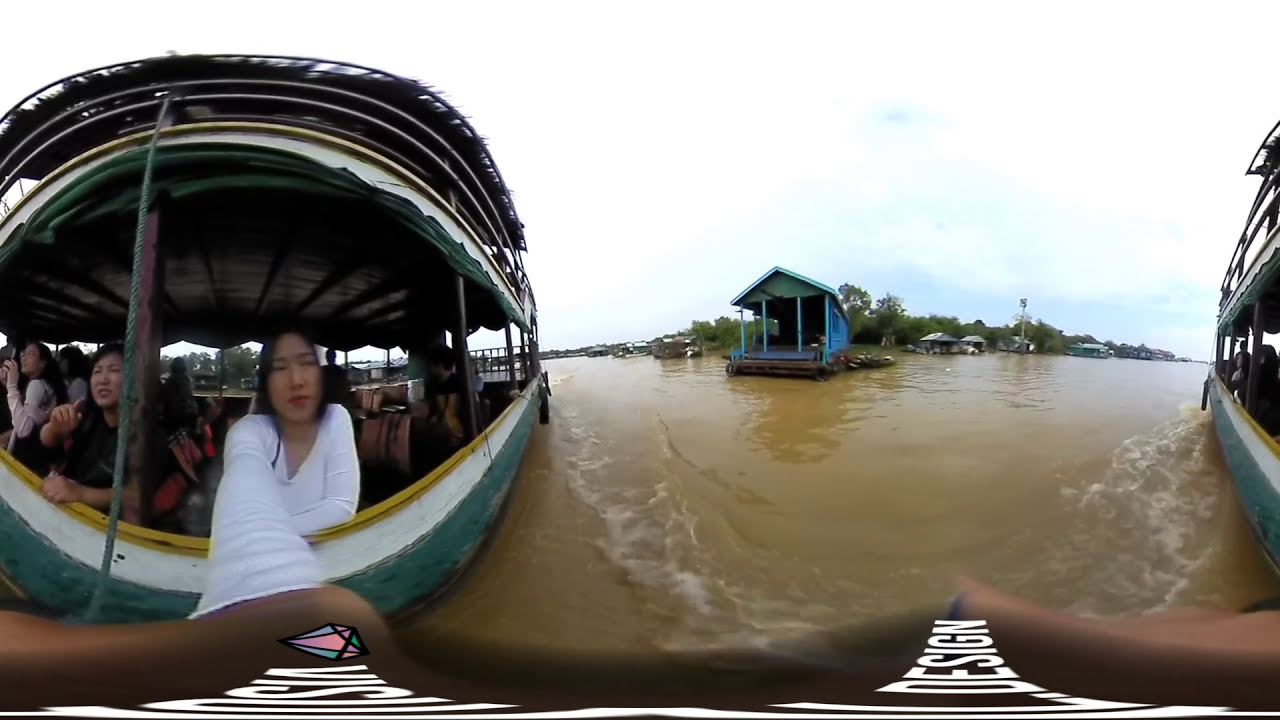This photograph captures an immersive 360-degree view of a group of Asian individuals on a small circular boat with a distinctive teal and white rim at the base, topped with a golden trim. The boat sits in murky, muddy brown water, surrounded by lush greenery and small huts on the riverbank in the background. The sky is light blue with scattered white clouds.

Prominently featured is an Asian woman in a white top, extending her arm over the side of the boat, holding the camera for a panoramic selfie. Her arm stretches across the bottom part of the image, which distorts the view, giving the impression of mirrored boats on either side. The right side of the image shows part of the boat along with some text, including the word “design,” partially visible at the bottom. A pink, green, blue, and purple diamond graphic is also noticeable at the bottom of the photo.

In the center of the image, there is a blue houseboat with a slanted roof. The boat has open windows and seating inside, and several other people can be seen on board, some capturing their own moments. The scenery features an assembly of trees and smaller buildings along the waterside. The boat generates white waves, enhancing the sense of movement in this dynamic riverscape.